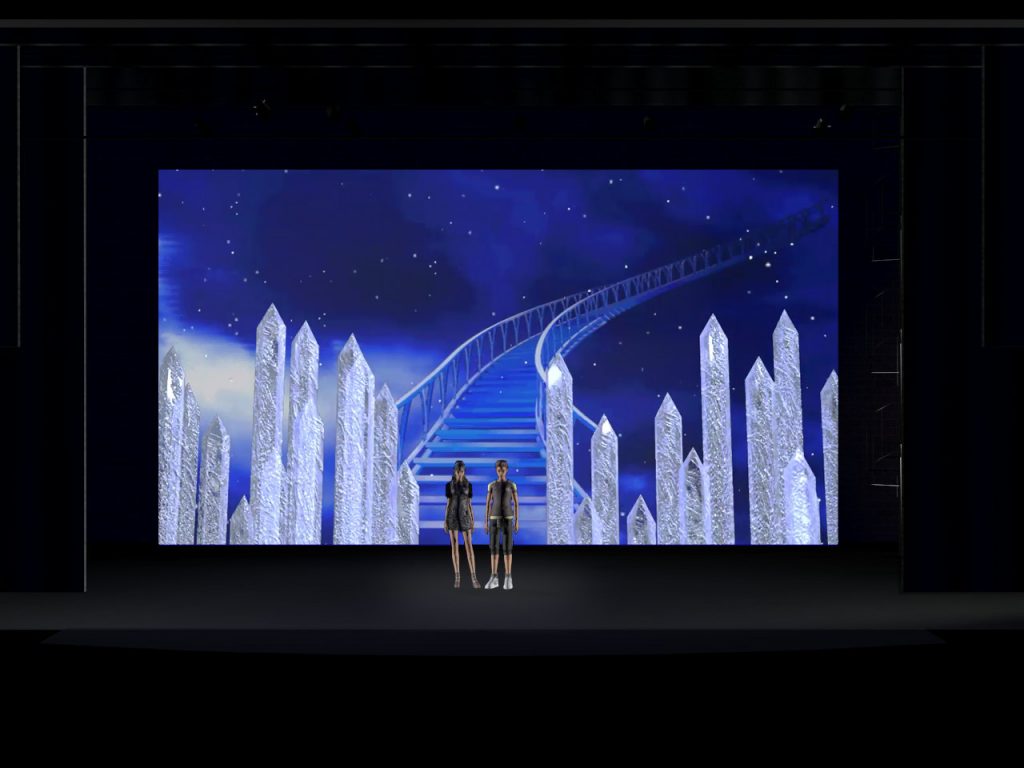In the computer-generated image, two young individuals, a male and a female, stand on what appears to be a dark stage, illuminated only by a large, vibrant screen behind them. The female, positioned on the viewer’s left, is dressed in a dark gray dress and has long brown hair. The male, standing to her right, is wearing knee-length pants, white sneakers, and a gray t-shirt. Both figures are facing the camera. The screen behind them displays a surreal, digital landscape dominated by shades of blue. Prominent in this background are large, white crystallized structures resembling icicles, flanking a central staircase that ascends into an ethereal night sky filled with numerous stars. The overall scene evokes a sense of being in a theater with the lights dimmed, creating a sharp contrast between the vivid digital imagery on the screen and the surrounding blackness of the stage.